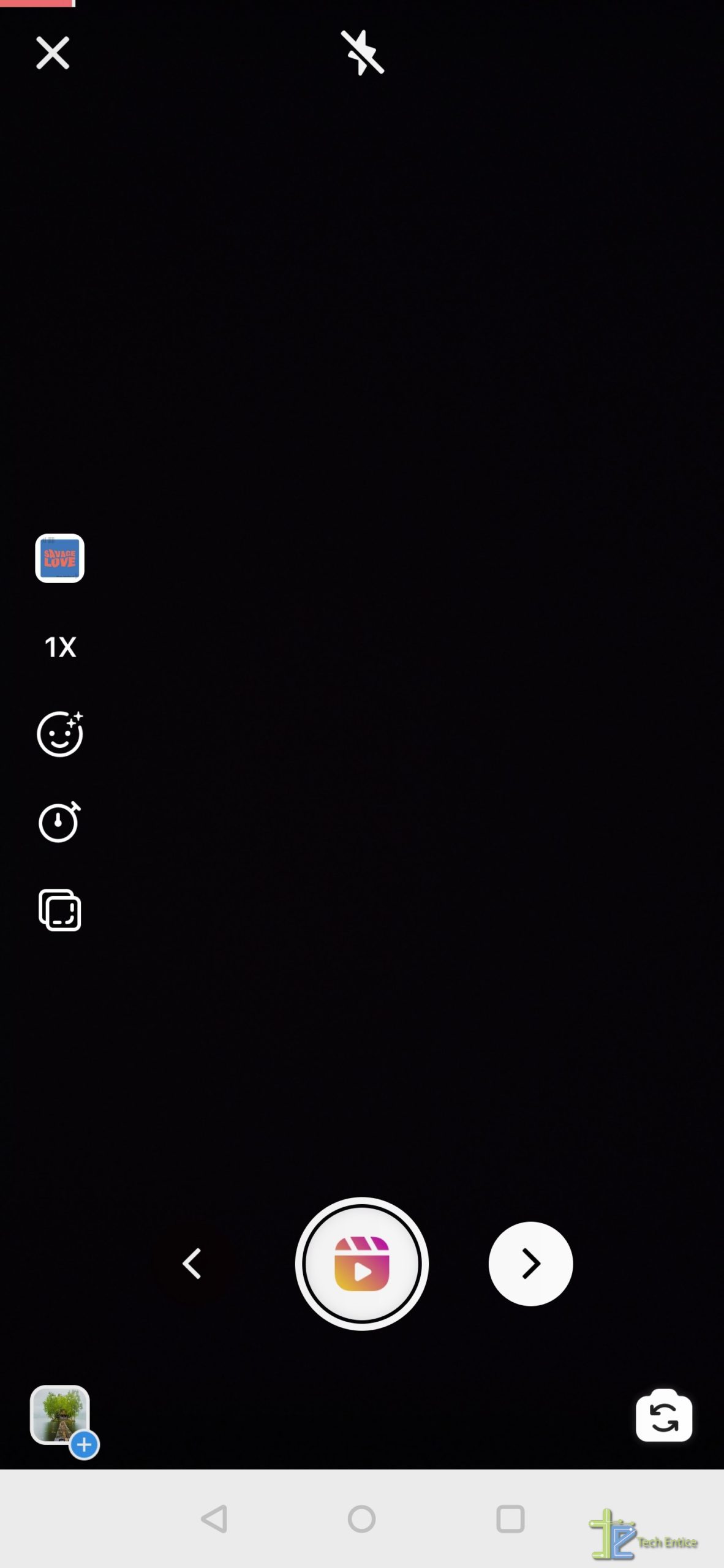The image depicts an iPhone with a black screen, positioned against a blue background adorned with red scribbles. At the top of the screen, there's a black bar, and particularly in the upper left corner, a red icon with an 'X' underneath suggests that the sound may be muted. The screen is predominantly dark, with a white-outlined box on the left side. Inside this outlined box, there are various icons: a '1x' indicator, a smiley face, a clock-like symbol, and two overlapping squares.

At the bottom of the screen, a prominent white circle features a complex icon resembling a box with three smaller boxes inside. This icon also includes a white triangle and arrows pointing left and right. The left side of the circle contains a green and brown square, while the right side has a blue circle with a plus sign. Additionally, there is a camera icon positioned at the bottom right corner of the screen.